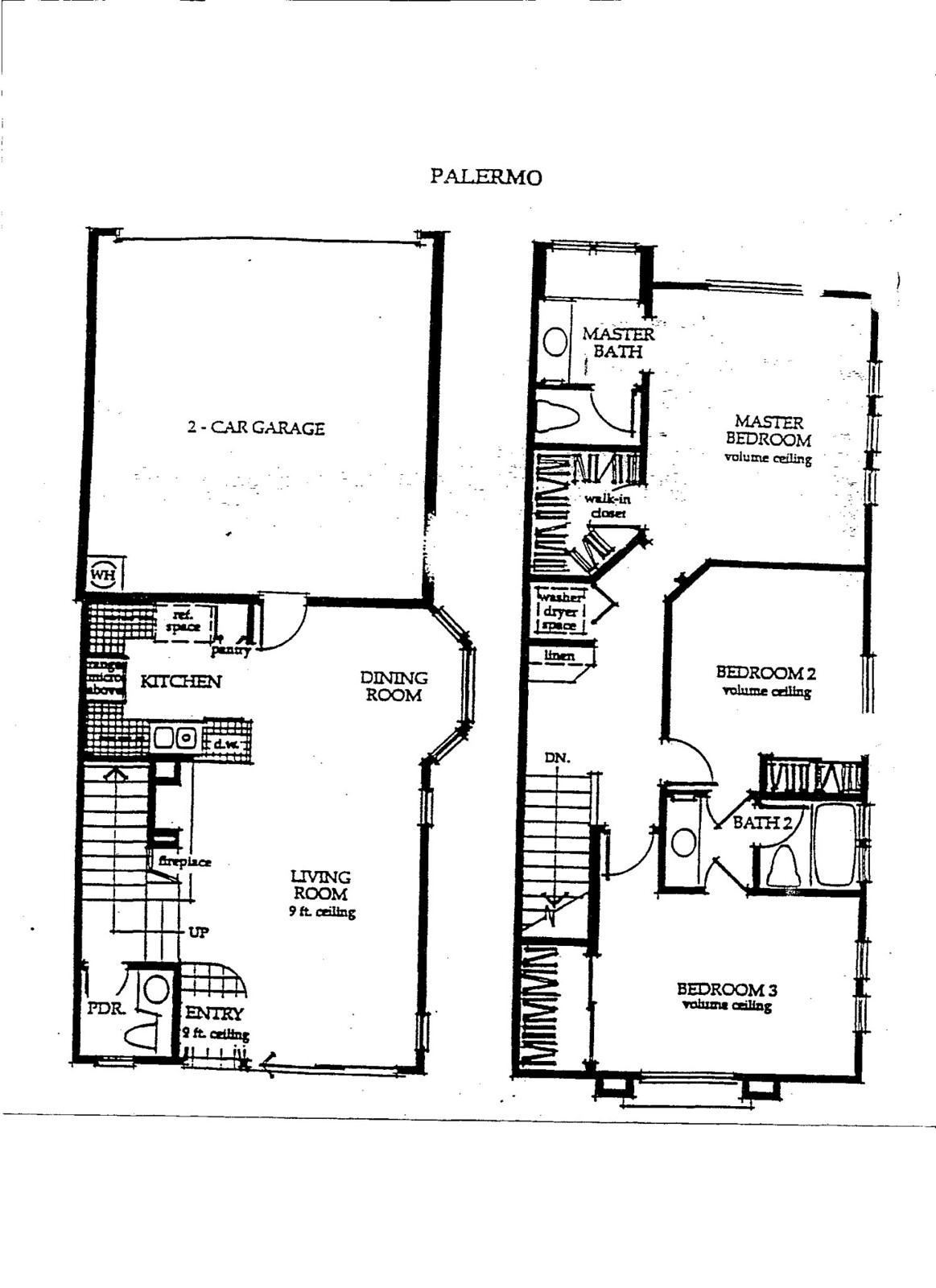This black-and-white blueprint outlines the detailed layout of a house styled as the "Palermo." Starting from the left-hand side, the image features a two-car garage marked with a square labeled "WH" and arcs on the top and bottom. From the garage, you enter the ground floor of the house, beginning with the kitchen that includes a pantry, space for a microwave and range, and a visible sink area. 

The open-plan design seamlessly connects the kitchen to the dining room, which then flows into the living room. The living area includes a fireplace, an entryway with an eight-foot ceiling, and a small powder room to the left. A staircase near the fireplace leads to the second floor.

Upon reaching the second floor, you find yourself in a hallway. Turning right takes you to Bedroom 3, which is adjacent to a bathroom complete with a sink, bathtub, and shower. This bathroom also has a door that connects to Bedroom 2, which features a volume ceiling. Accessing Bedroom 2 directly from the hallway is also possible.

Continuing down the hallway leads to the master bedroom, which also boasts a volume ceiling. Attached to the master bedroom is a master bath equipped with a toilet, sink, tub, and shower, as well as a spacious walk-in closet.

Additionally, the second floor includes a designated space for a washer and dryer, along with a linen closet, conveniently located in the hallway.